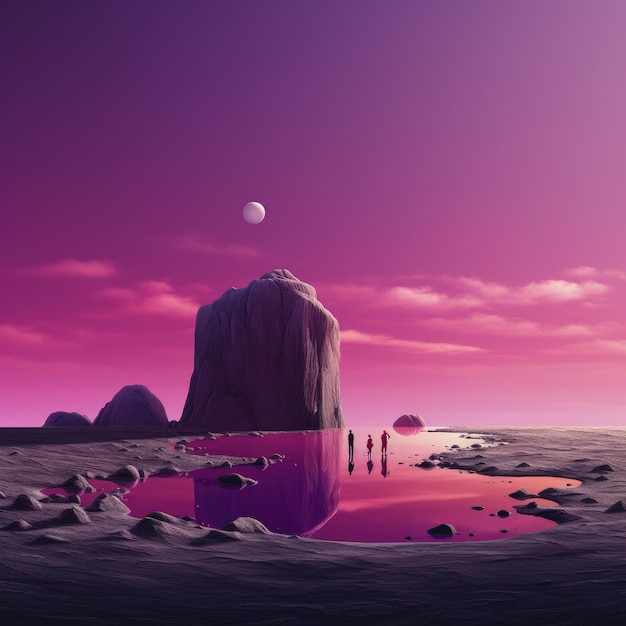The fantasy image depicts a strikingly surreal landscape under a mystical, deep purple sky that transitions into a vibrant pinkish-magenta near the horizon. White clouds dot the sky, adding to the otherworldly atmosphere. A full, luminous white moon hangs prominently in the distance. The scene features a large, central square-shaped rock formation flanked by two smaller hills to its left. In the foreground, the rocky and uneven ground suggests a muddy beach, with black sand extending toward the water. This body of water mirrors the enchanting colors of the sky, enhancing the magical aura of the scene. Intriguingly, three figures—two taller and one shorter—are seen standing in the water, possibly a family, though their exact relationship remains ambiguous. The overall sharp, detailed quality of the image suggests it may be a digitally created artwork, capturing a vivid, dream-like world.